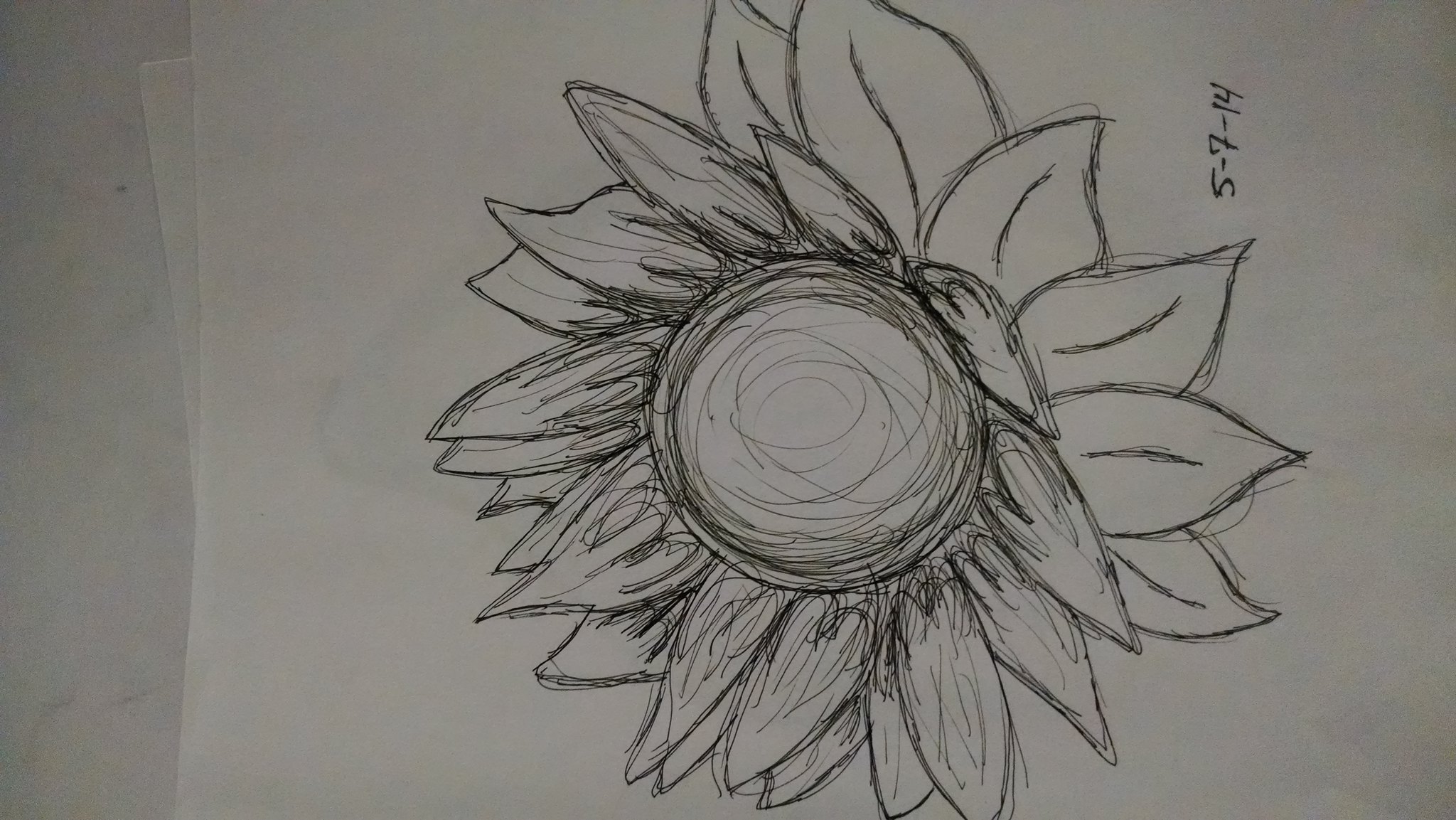This image features a detailed pen sketch of a flower that resembles a sunflower, prominently positioned on the left side of the frame after being rotated 90 degrees sideways. The sketch captures the essence of a sunflower with its petal shapes, though the center deviates from typical seed patterns, displaying a series of intricate, spiral-like outlines instead. The sketch is rendered on a pristine white piece of paper. In the top right corner, the date "5-7-14" is inscribed, indicating when the artwork was completed. Additionally, a partial view of another piece of paper can be seen peeking out from the top of the image.